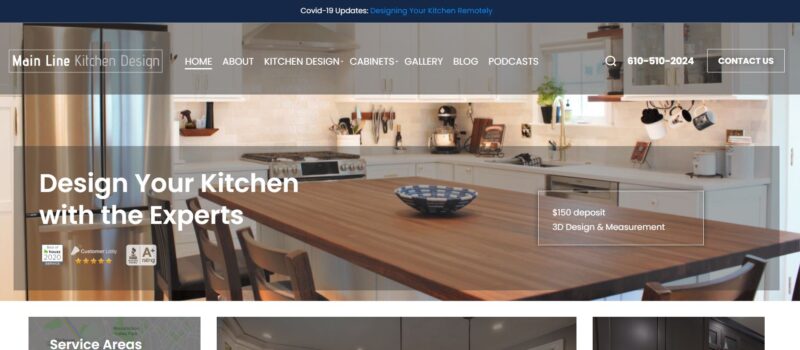The image captures a sophisticated kitchen design promotional layout. At the top of the image, a refined navy border frames white text mentioning "COVID-19 Updates" alongside a blue message stating "Designing Your Kitchen Remotely." Below this section is a visual background of a modern kitchen scene featuring elegant countertops and a sizable table. Overlaid on this background are menu options at the top, including "Me in Line Kitchen Design," "Home" (currently selected), "About," "Kitchen Design," "Cabinets," "Gallery," "Blog," "Podcasts," and additional icons like a search icon, telephone number, and a "Contact Us" button.

Beneath the navigation menu, bold white lettering on the left declares “Design Your Kitchen with the Experts.” Below this, various icons emphasize accreditations and customer reviews, validating the quality of the kitchen designs. On the right side of the image, a transparent box overlays the table area, detailing a promotion that includes a "$150 Deposit," "3D Design," and "Measurement."

At the very bottom of the image, several additional pictures are visible, with one on the left highlighting "Service Areas." The overall composition combines a sleek, professional aesthetic with informative elements designed to engage potential clients.